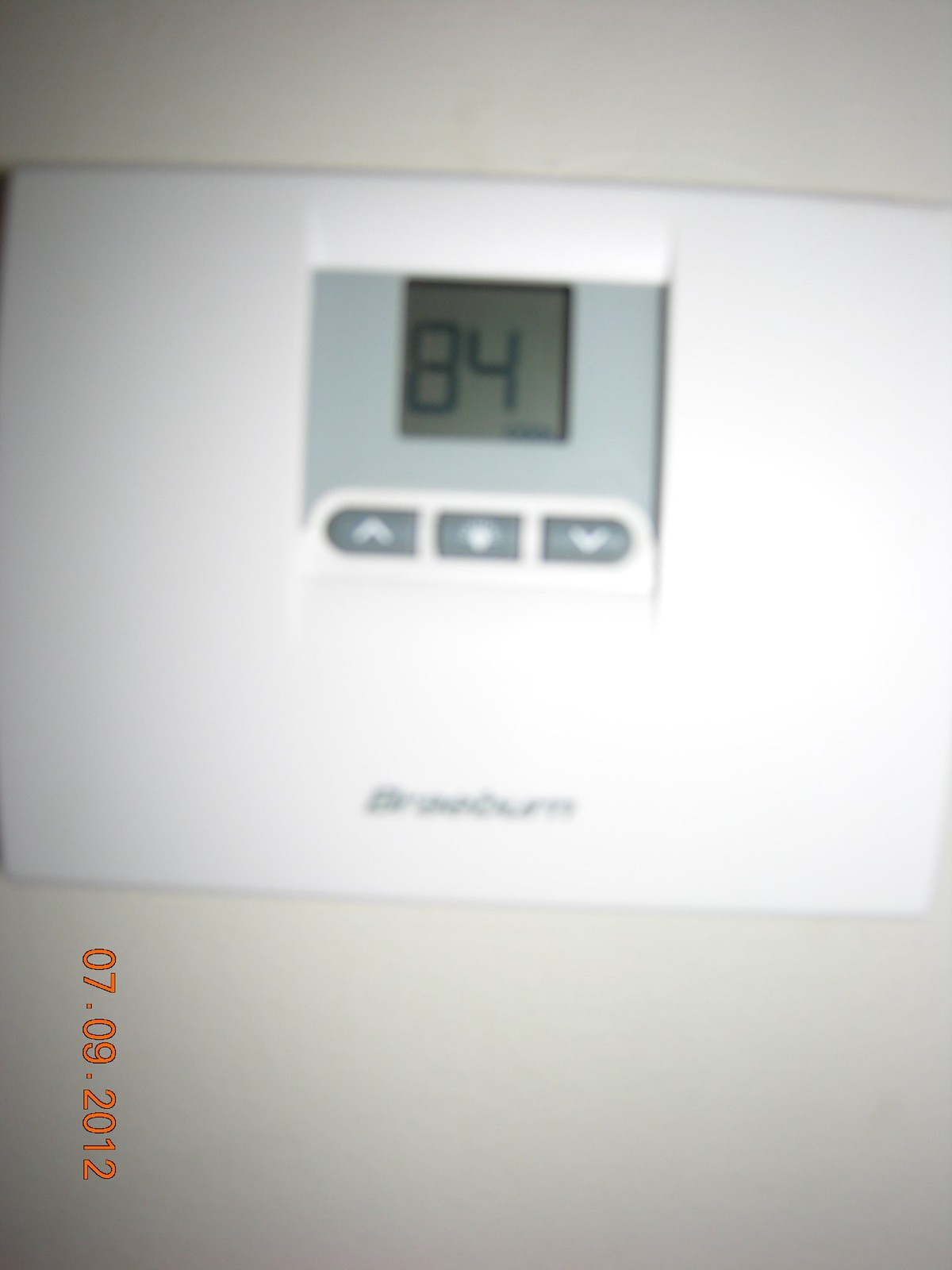This image showcases a somewhat blurry bathroom scale positioned against an off-white backdrop, which appears to be the scale itself. The scale features a rectangular display panel at the top, capable of showing weight measurements up to three figures. Although the display is out of focus, it currently indicates a weight of "84." Beneath the display, there are buttons likely intended for adjusting the settings or calibration of the scale. In the bottom left-hand corner of the image, the date "07.09.2012" is displayed vertically, suggesting the photo was taken either on September 7th or July 9th, 2012. Due to the blurriness, the brand name on the scale remains illegible.